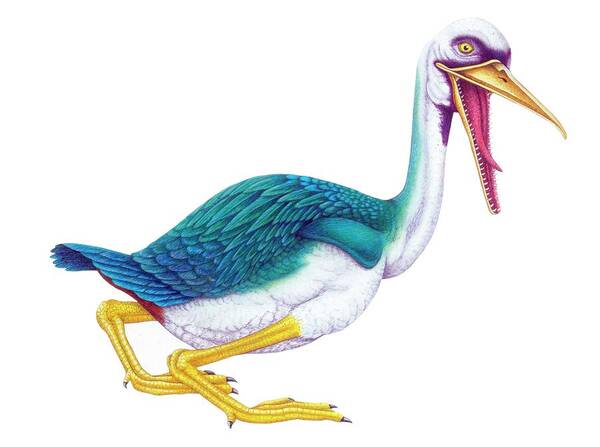This highly detailed, color illustration features a hybrid bird with the body of a duck. Its predominantly white feathers are accented with greenish-blue on its back. The bird has a long neck reminiscent of an ostrich's and two long, yellow legs adorned with sharp, black talons. Its large, pointed yellow beak is open, revealing menacing zipper-like razor-sharp teeth and a long purple tongue. The bird's face is uniquely colored, with a mix of yellow eyes, purple around the front, and yellow legs. The strikingly detailed drawing appears to be created with markers, colored pencils, or watercolor and is set against a plain white background, enhancing the unsettling and eerie appearance of this fantastical creature.